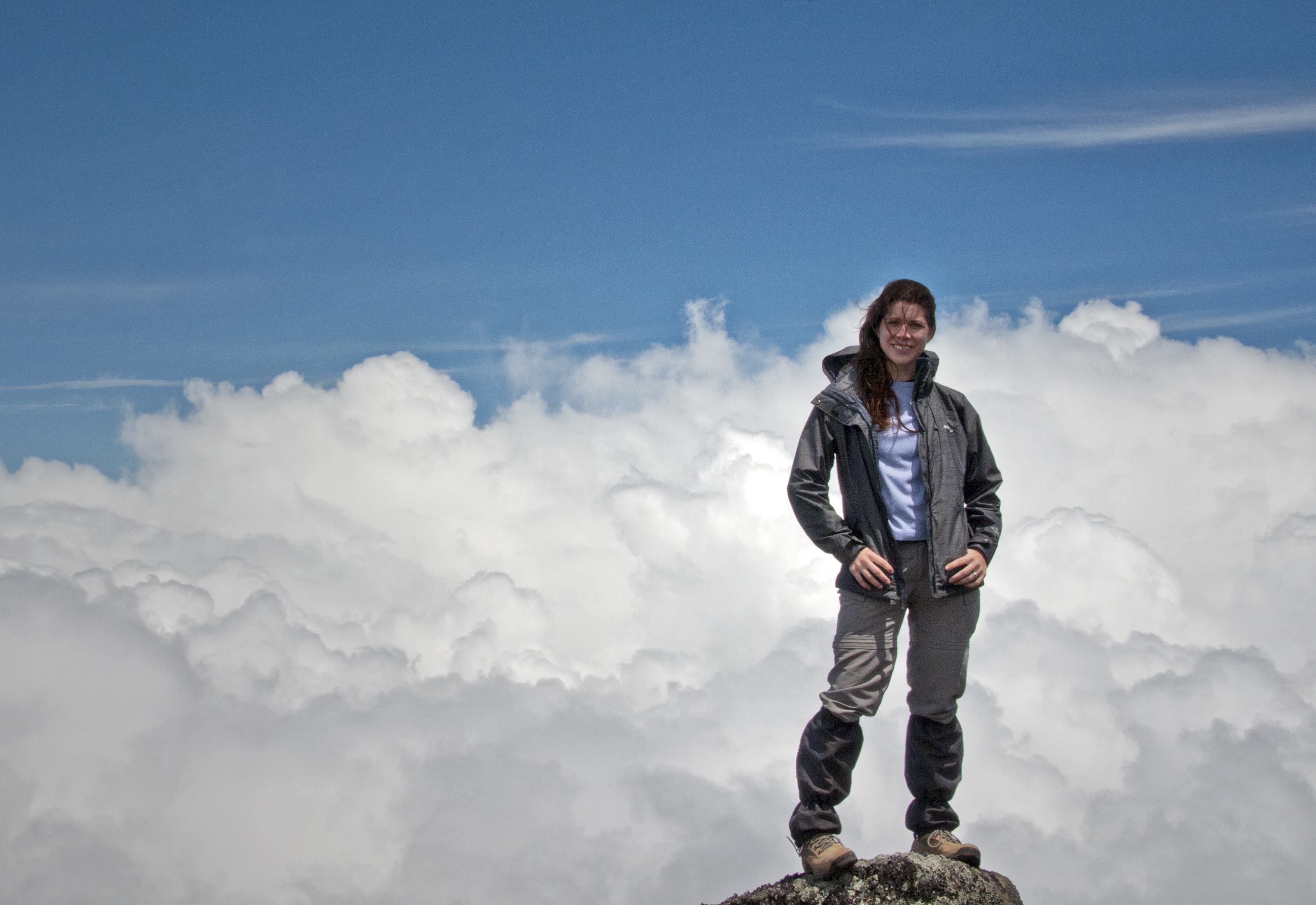A woman stands triumphantly atop a boulder, only the very tip of which is visible at the bottom of the image, giving a sense of her lofty perch. The backdrop reveals a breathtaking view, with clouds drifting below her, indicating her high elevation, likely at the summit of a mountain. Beyond the clouds, the clear sky stretches infinitely. She is dressed in an unzipped jacket over a blue shirt, complemented by light and dark gray hiking pants and sturdy hiking boots. Her relaxed stance, with thumbs tucked into her jacket pockets, and her brown hair casually draped over one shoulder, embody the spirit of adventure and achievement.